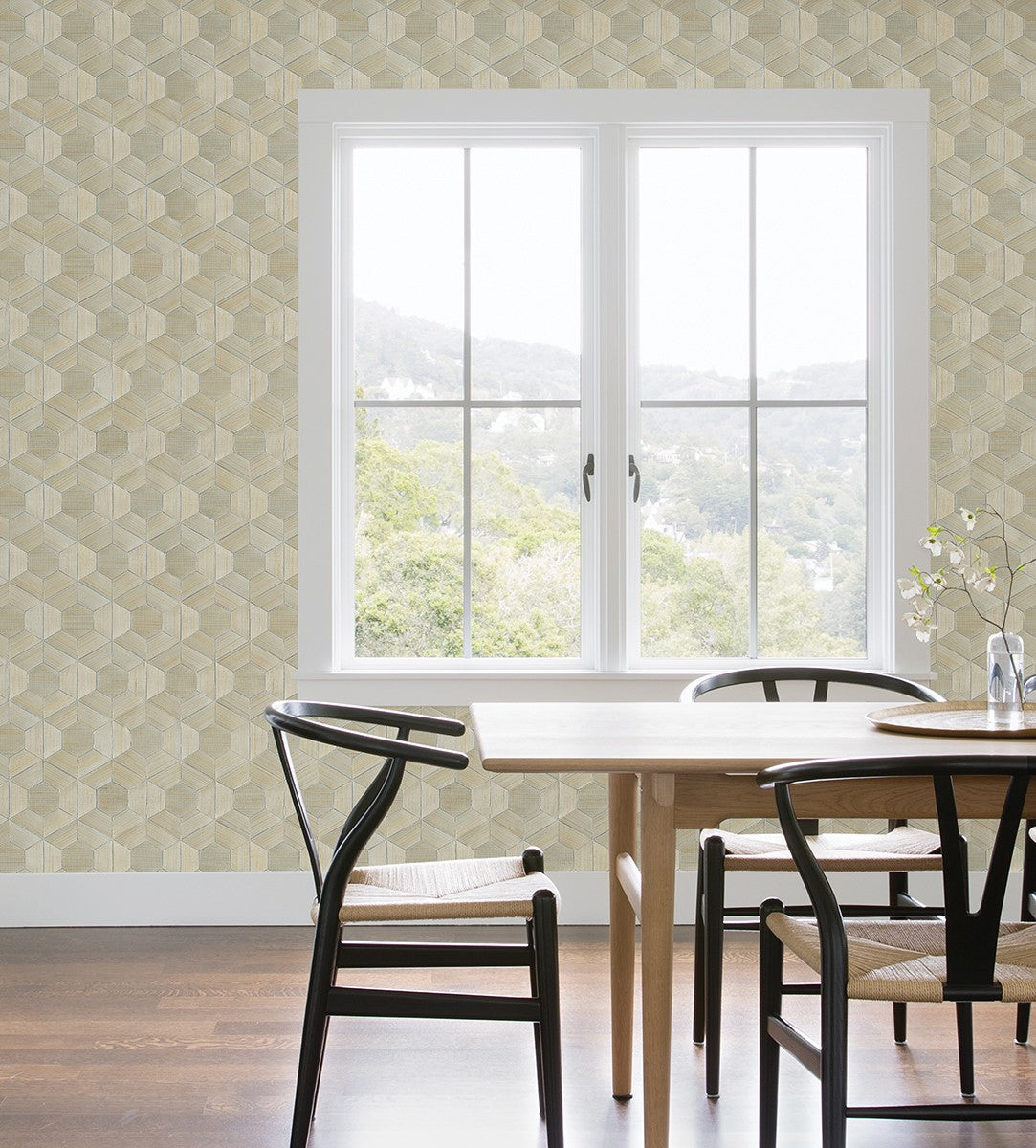The image depicts an early morning dining scene in an airy, light-filled dining room. At the center of the room is an oak dining table, which is tan in color and complemented by three visible metal chairs. These chairs feature short, rounded backs and seats crafted from tan rattan. Positioned behind the table, a large picture window frames a scenic view of a hilly, tree-covered landscape, abundant with heavy vegetation, valleys, hills, and a visible skyline. The window, devoid of curtains or blinds, is trimmed in white and equipped with two handles for opening. The dining room's wallpaper is bold, featuring an octagonal rattan pattern in a tan or beige hue, adding texture to the setting. On the table sits a platter adorned with a tall clear vase containing a branch with flowers, bringing a touch of nature indoors. The room's floor is a dark hardwood, complete with wide base trim. The combination of modern and natural elements creates a refreshing and picturesque dining environment.